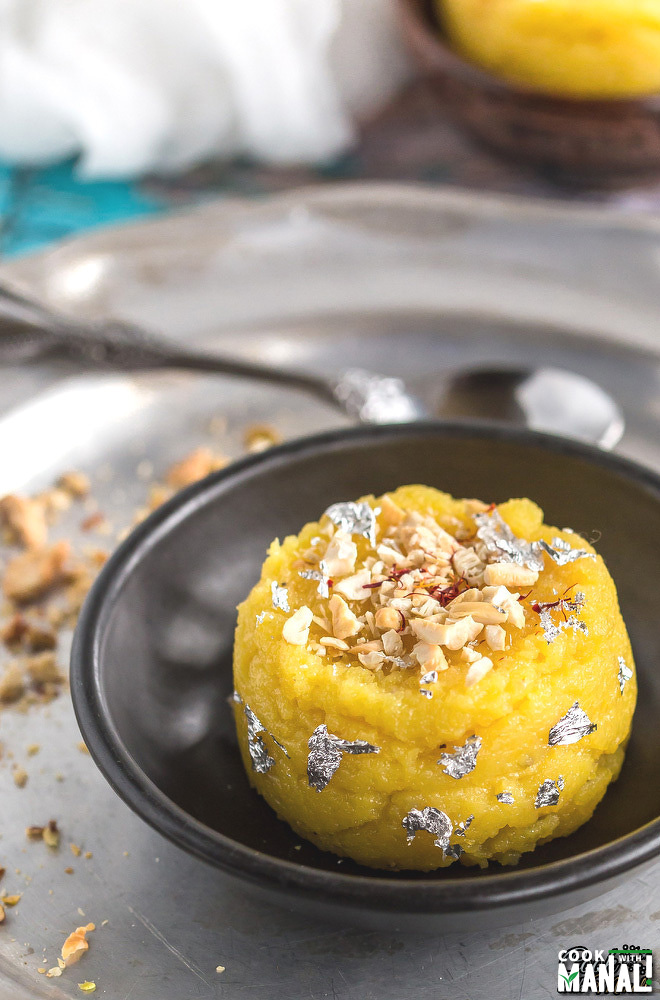This close-up photograph showcases a small, intriguing yellow cake-like pastry delicately nestled in a small black bowl. The pastry, which might be fruit-based, boasts a unique appearance with its yellow hue and an outer layer adorned with edible silver flakes, reminiscent of tinfoil. Atop the pastry, a generous sprinkling of crushed nuts, possibly walnuts, adds texture and contrast. This black bowl is arranged on a silver tray that bears the remnants of the sprinkled nuts and crumbs, hinting at previous indulgences. In the background, slightly out of focus, a spoon rests on the tray, and another bowl containing a similar pastry is faintly visible. The bottom right corner of the image displays the logo "Cook with Manali," anchoring the composition and hinting at its culinary origin.